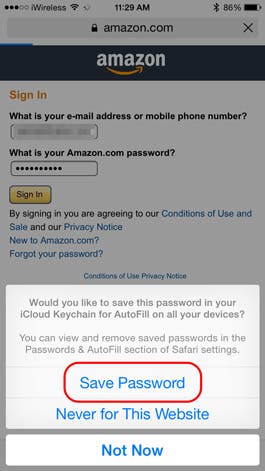The image displays an old Amazon sign-in page viewed on a smartphone. The phone's status bar, centered at the top, shows the time as 11:29 a.m., a battery life indicator at a critically low 6%, a Bluetooth icon, and a Wi-Fi signal symbol. Below this, the Amazon search bar is visible, followed by the recognizable Amazon logo.

The focus is on the sign-in form, which prompts the user with fields for their email address or mobile phone number and their Amazon password, the latter of which is obscured by password dots. A yellow "Sign In" button is prominently displayed beneath these fields. Under this button, a message states, “By signing in, you are agreeing to our Conditions of Use and Sale and our Privacy Notice.” The page also includes options for users new to Amazon and those who have forgotten their passwords, with clickable blue links allowing further navigation.

A partially open iCloud Keychain prompt appears at the bottom, asking, “Would you like to save this password in your iCloud Keychain for autofill on all your devices? You can view and remove saved passwords in the Passwords & Autofill section of Safari settings.” The options presented are “Save Password” (highlighted with a red box), “Never for This Website,” and “Not Now,” all in blue text. The red box around "Save Password" indicates the user's intention to save their Amazon login information for future ease of access.